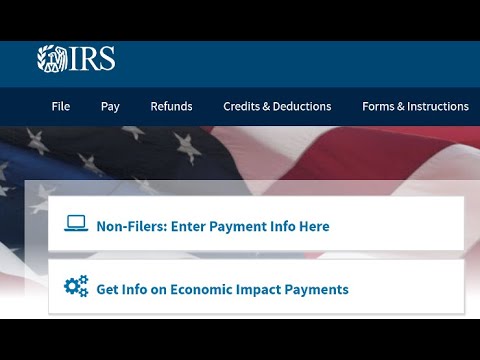The image shows an IRS webpage with a prominent black banner at both the top and bottom of the page. The top of the page features a blue background, while the middle section displays a waving American flag. The IRS logo is visible, featuring a scale and leafy branches on the left, and a feather-like motif on the right. Most of the text is written in white, including key terms like "File," "Pay," "Refunds," "Credits and Deductions," "Forms and Instructions," all of which are displayed prominently. Information for non-filers to enter payment info and details on economic impact payments is also highlighted. The rest of the text is blue and is framed by a white background box providing clear contrast and readability.